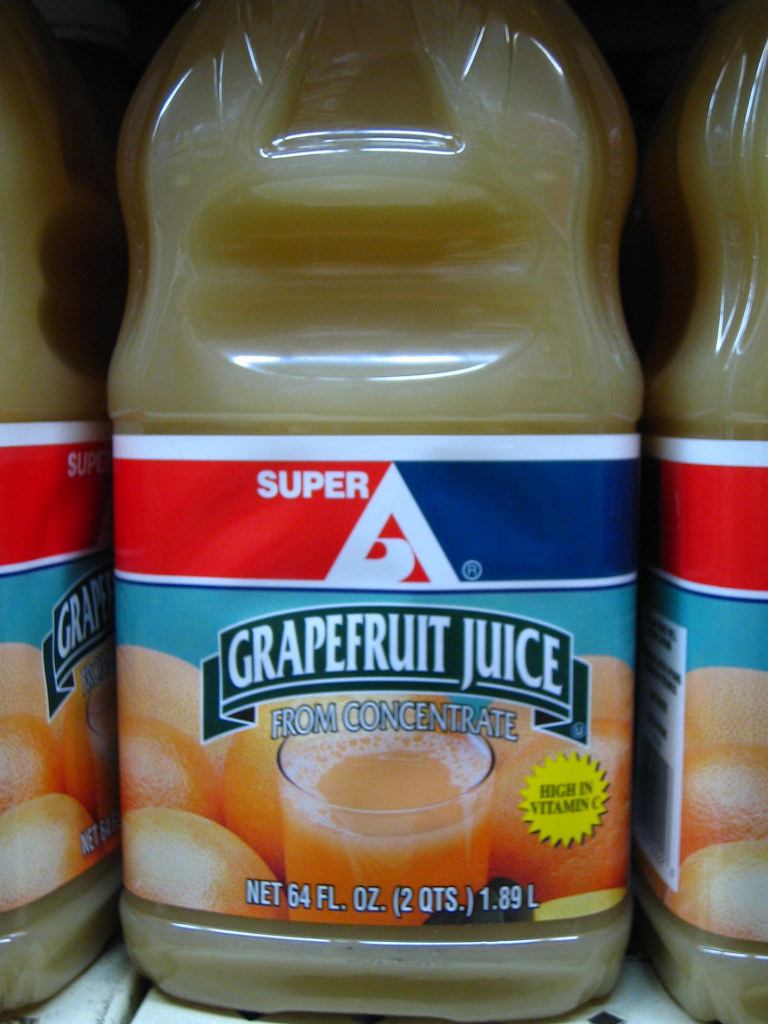The image captures a prominently displayed plastic bottle of grapefruit juice positioned on a shelf within a grocery store. The top portion of the bottle is cut off, leaving the cap out of view, but the main body of the bottle remains clearly visible. The label on the bottle boldly reads "Grapefruit Juice" and mentions that it is "from concentrate." A vivid illustration on the label features a full glass of grapefruit juice surrounded by whole grapefruits, visually emphasizing the fresh and tangy flavor. Additional text on the label highlights that the juice is "High in Vitamin C," promoting its health benefits. Flanking the featured bottle on both the left and right are other similar bottles, lined up neatly on the shelf, indicating a well-stocked section dedicated to grapefruit juice in the store.